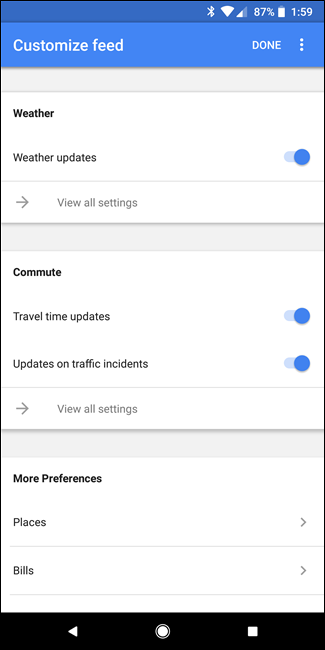In this smartphone screenshot, the scene is framed by a black outline, indicating the edges of a phone display. At the very top, a dark blue status bar displays essential information: a battery icon showing 87% charge and the current time of 1:59, along with a Wi-Fi signal indicator positioned to the left of the battery percentage.

Below the status bar, a lighter blue rectangular banner spans across the screen, displaying "Customize speed" in white text, with the word "Done" and an ellipsis symbol (three white dots) to its right, suggesting further options upon interaction.

The next section is a white background, organized into clearly defined areas. In the upper left corner, the word "Weather" stands out, followed by a noticeable gap. Below this, "Weather updates" is written alongside a blue toggle button to indicate that the updates feature is currently activated.

Proceeding further down, another white area contains the text "View all settings," acting as a link for additional configurations. A narrow gray bar separates this section from the one below.

The next white rectangle is labeled "Commute" at the upper left. It presents two toggled options: "Travel time updates" and "Updates on traffic incidents," both with active blue toggle buttons. Below these options, a "View all settings" link is again provided for extended adjustments.

After another gray divider, the final white rectangle is titled "More preferences." This section offers additional adjustable options labeled "Places" and "Bills," rounding out the detailed menu of customizations available on this screen.